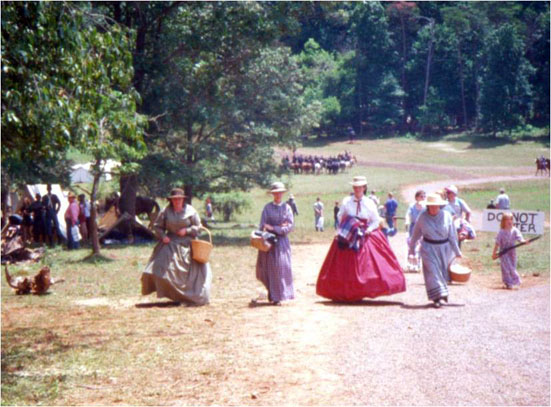The image appears to be a vibrant, colorized photograph from the late 1800s or early 1900s. It captures a lively gathering amidst a backdrop of verdant, light green trees. Central to the scene are four women dressed in period attire. Their outfits are ornate and reflect the fashion of the era. One woman stands out in a dress that features a white bodice adorned with a striking red ribbon around her neck. Each woman is accessorized with a beige hat, adding to the historical ambiance. The skirts or dresses, particularly one that is notably fluffy and red, enhance the vintage feel. In the background, additional figures are present, though their identities and actions remain indistinct even upon closer inspection. The scene evokes a sense of nostalgia, offering a window into a bygone time of social gatherings and elegant attire.